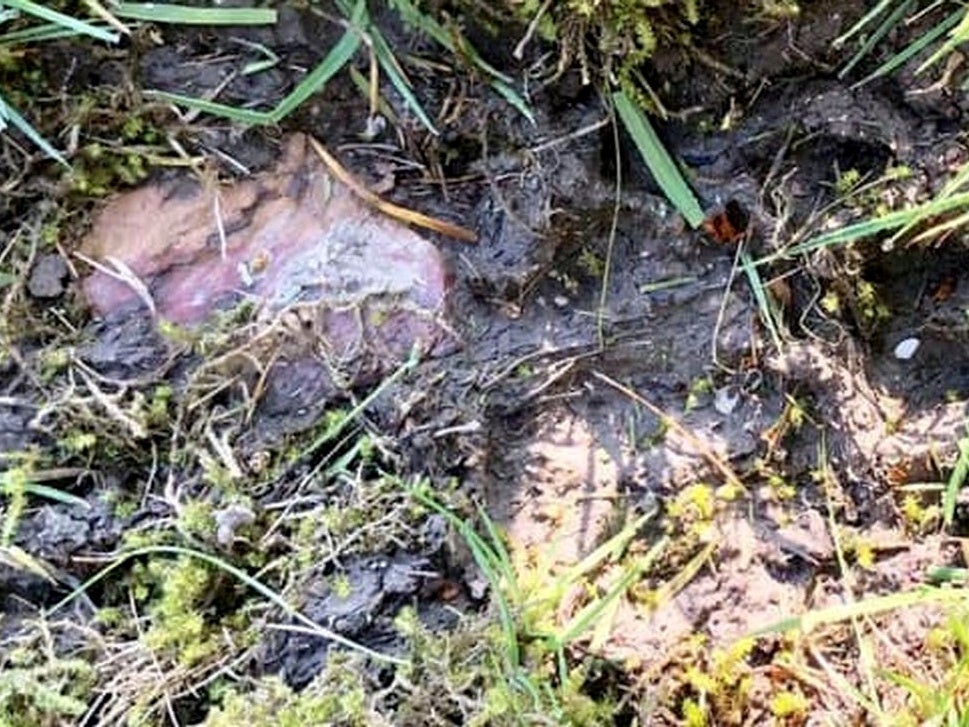This photograph captures a small, earthy section of ground, predominantly characterized by its wet, muddy texture. The central portion of the image is dominated by dark, blackened mud, interspersed with blades of grass that emerge sporadically, even at the top of the area. The bottom of the image features shreds of grass and moss, mingling with a beige-colored, relatively drier patch of soil. Off to the bottom right, the ground appears less saturated, suggesting a transition from the slick, tan soil to the more absorbent dark brown mud above it. On the upper left, there is a notable rock with beige and purple striations, caked with gray mud. Scattered across the scene are yellow flowers and small bushes, adding speckles of color to the otherwise earthy tones. The composition hints at natural disturbances, resembling uprooted tree stumps, with circular impressions hinting at their previous presence. Overall, the photograph presents an intricate tapestry of muddy, earthy textures enriched with varied vegetation and subtle natural elements.